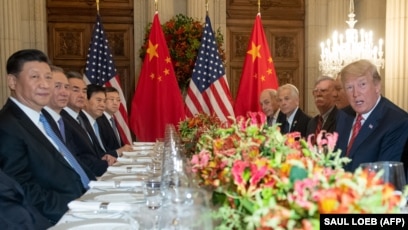This photograph captures a formal state dinner held during Donald Trump's presidency, featuring an official meeting between United States and Chinese representatives. Seated at an elegantly set table with white tablecloths and napkins, Donald Trump is positioned on the right-hand side, engaging with the camera and appearing to be in mid-sentence. To Trump's right are four American men, all dressed in suits, while across the table sit five Asian men, equally formal in their attire. A stunning floral centerpiece, bursting with vibrant colors, adorns the middle of the table, which is set with plates, glasses of water, and neatly arranged place settings, though the meal has not yet begun. The background of the room is adorned with flags from both nations—two American flags interspersed with two red flags bearing gold stars, indicative of China. This formal setting is further accentuated by a grand, well-lit chandelier hanging prominently behind Trump's head. Most participants are looking toward the camera, capturing the gravity and formality of the event. The photo acknowledgment credits Saul Loeb of AFP.